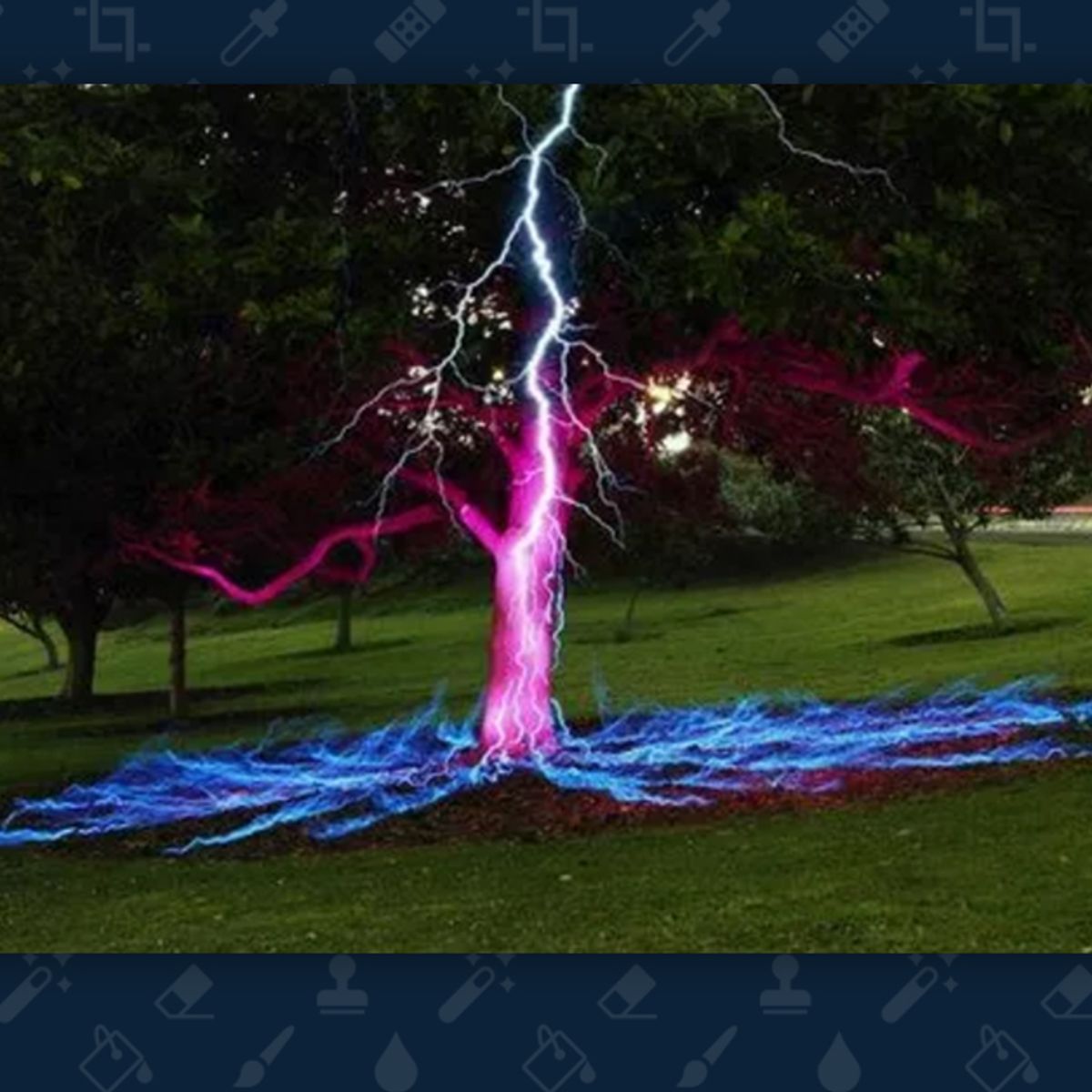This professionally captured, full-color, vertical nature photograph primarily showcases a dramatic scene of a lightning strike hitting a tree in the middle of a lush park. The composition is clear and detailed, with a blue border at the top and bottom of the image. Various medical-themed watermarks, like eyedroppers, band-aids, nurses, and doctors, are scattered across the photo.

The central focus is the lone tree struck by a vivid bolt of lightning, with the white lightning striking the top and transitioning to a striking purple as it makes contact with the trunk and branches. This purple hue permeates the tree's structure, extending from the trunk into the branches. Below, at the root system, the lightning spreads out above the ground, creating an eerie, glowing, fiery blue effect that adds to the mystical aura of the scene. Surrounding the highlighted tree, you can see a rich green grassy field and several other trees in the background, their leaves a deep forest green. The blend of natural and intense colors—green, purple, bright pink, and various shades of blue—adds to the captivating and somewhat surreal atmosphere of the photograph.